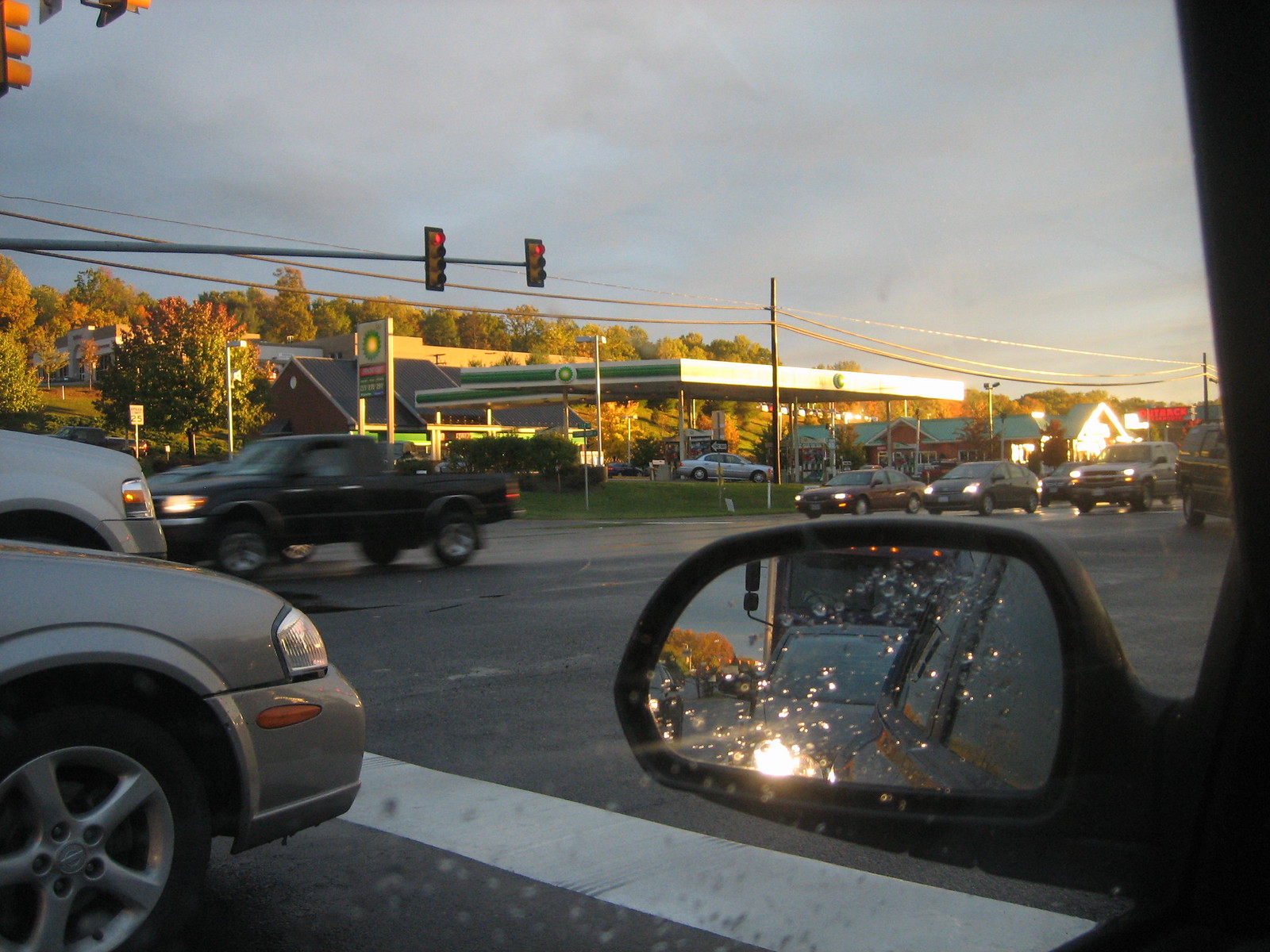This photograph captures a moment on the road either just before sunset or just after, likely following a recent rainstorm. Taken from within a car, the side mirror is visible, showing raindrops that haven't yet dried, hinting at the recent weather. Reflections of other vehicles can be seen in the mirror. The scene is at a crossing where traffic lights signal and cars move along the opposite side. Dominating the foreground is an SBP gas station, illuminated by soft evening light breaking through the dim, gray sky. The sky remains overcast, but the emergence of sunlight to the right signals the storm's end.